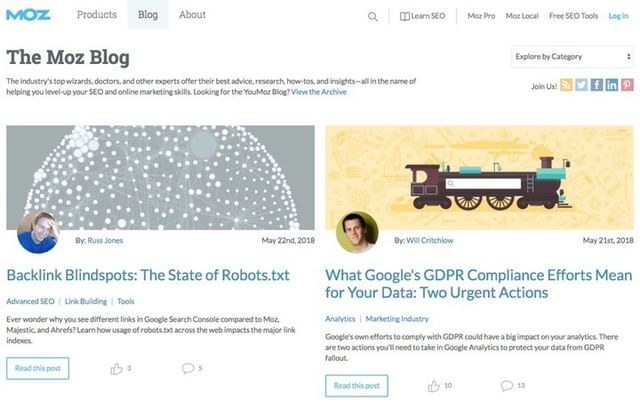In the top left corner of the image, there is a blue logo that reads "MOZ." The title bar spans across the top and includes the options "Products," "Blog," and "About." On the right side of the title bar, there is a small search icon. Below this, navigation links read "Learn SEO," "Moz Pro," "Moz Local," "Free SEO Tools," and "Log In."

The main heading is "The MOZ Blog." Directly beneath this heading, a paragraph reads: "The industry's top wizards, doctors, and other experts offer their best advice, research, how-tos, and insights, all in the name of helping you level up your SEO and online marketing skills. Looking for the UMOZ blog? View the archive." 

Below this text are two side-by-side sections. The left section is titled "Backlink Blind Spots: The State of Robots.txt." The right section is titled "What Google's GDPR Compliance Efforts Mean for Your Data: Two Urgent Actions," accompanied by a graphic illustration of a train above the respective titles. Each section has a round profile photo above its title, presumably of the article authors.